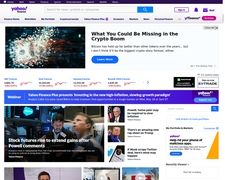This cropped screenshot captures a portion of the Yahoo front page, showcasing its distinctive layout. The page features a clean white background. At the top left corner, "Yahoo" is prominently displayed in purple. Centered on the page is a search bar, accompanied by a blue box containing a white magnifying glass icon on its right side. The header also includes a series of categories set against a gray background, with another Yahoo logo situated at the far right.

Beneath the header, a large thumbnail image is present, adjacent to a bold black headline stating, "What you could be missing in the crypto boom." A concise description follows this headline, accompanied by a blue button that directs readers to the full story.

In the center, a horizontal ticker displays stock information. Below this ticker lies a substantial blue banner promoting a Yahoo advertisement. Below this advertisement, the page is divided into two columns: the left column features a large square photo with an overlaid text description, while the right column presents a vertically arranged list of smaller thumbnails and story headlines.